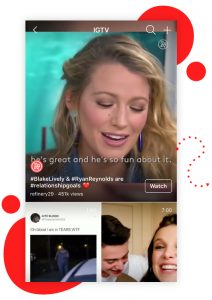This image depicts a cluttered Instagram screen with a notable white background adorned with intriguing red dots, providing a unique backdrop. At the top center, the IGTV logo is prominently displayed, suggesting this section contains a video, which indeed appears to feature Blake Lively. The video is labeled with hashtags such as #BlakeLively, #RyanReynolds, and #RelationshipGoals, accompanied by a heart emoji, indicating a focus on the star couple's relationship. 

Beneath this main content, a blurred meme is partially visible but unreadable, adding a touch of humor or commentary that remains elusive. Adjacent to the unseen meme, another video thumbnail features Millie Bobby Brown alongside a co-star from Stranger Things, enhancing the celebrity and pop culture theme.

The layout seems to be part of an Instagram feed or explore page and is visually striking with its novel arrangement, which diverges from traditional Instagram layouts. Dominating the screen, the Blake Lively video is the most highlighted element, equipped with a 'watch' button located at the bottom right corner, encouraging viewers to engage with the content.